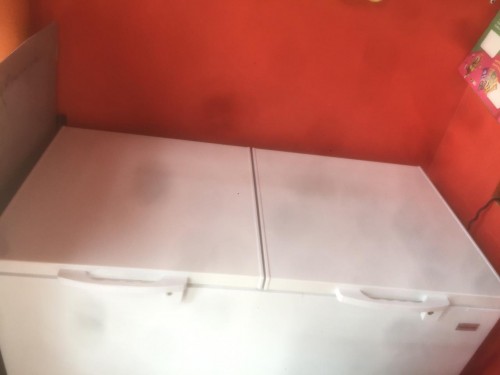In the image, there is a large, white deep freezer centered against a vibrant red or coral-colored wall. This deep freezer, which has two doors with white handles that lift upwards, shows some signs of wear and smudges on its surface. To the right of the freezer, a black power cord can be seen trailing up to a nearby outlet. On the wall above the outlet, there's a poster featuring cartoon characters, with green and pink segments, possibly adorned with post-it notes. Additionally, a small label is affixed to the lower right corner of the freezer, though the details on it are not legible. To the left of the deep freezer, a thin wall or separator is visible, emphasizing the room's layout.